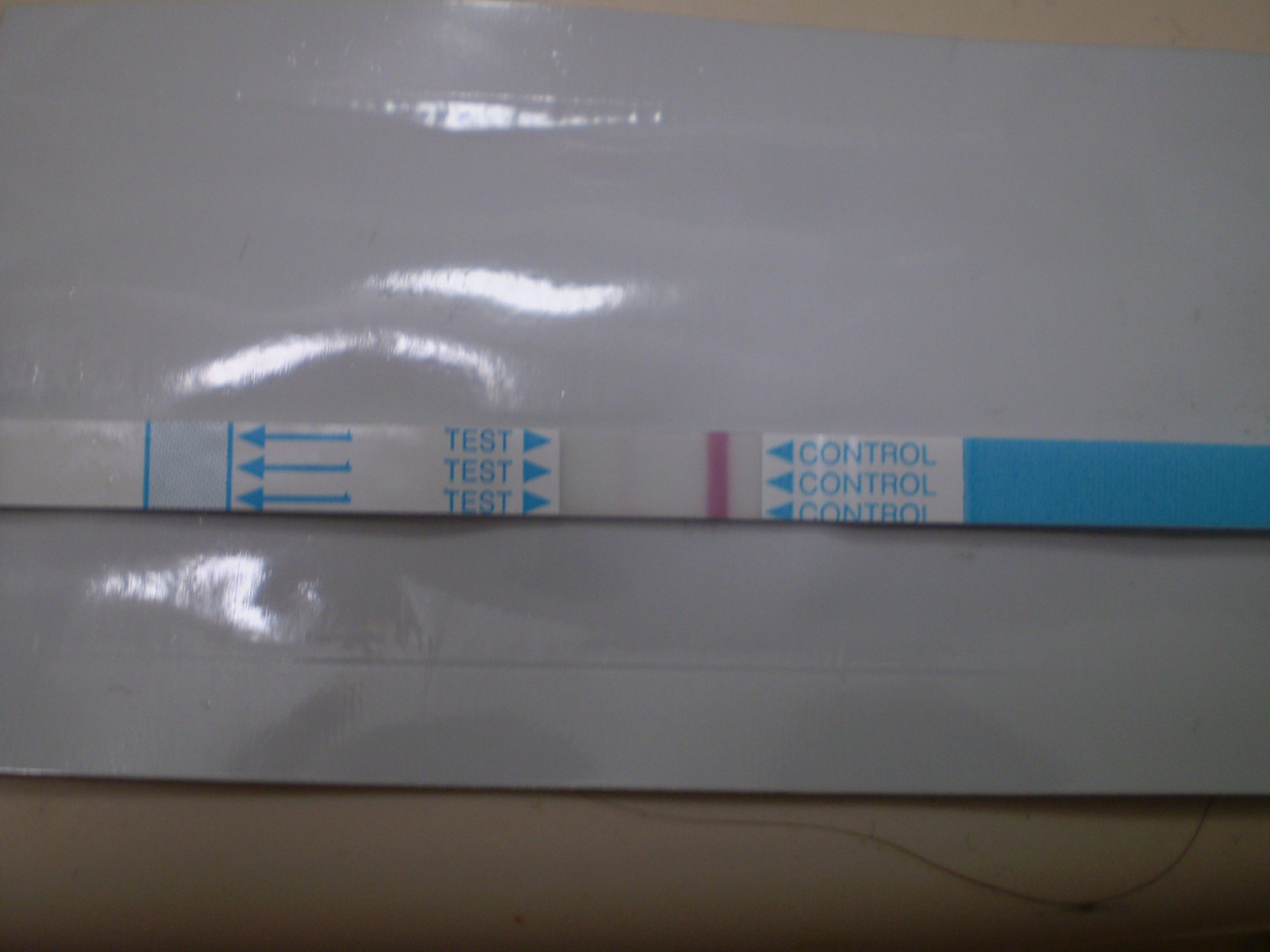This photograph captures a medical or chemical test strip used for determining water quality or other analytical purposes. The focal point is a narrow test strip that spans the entire width of the photograph, positioned centrally in terms of vertical alignment and resting on a shiny white surface, likely laminated paper or plastic. This white surface features four wave-shaped bright white highlight reflections on the left half of the image.

The white surface is positioned atop a barely visible, beige-colored background, seen as a thin strip along the upper right and the entire lower edge of the photograph. Adding a touch of realism, a thin black piece of thread or hair curves out from beneath the white surface.

The test strip itself is predominantly white and light blue, featuring a prominent vertical red bar. On the far right end, a solid blue section transitions to a white segment with the word "CONTROL" printed in light blue, repeated three times in a vertical stack. Adjacent to each "CONTROL" word, blue arrows point to the left, directing attention to the vertical red line. Next to the red line, another white section showcases the word "TEST" in blue, with an arrow pointing to the right and flanked by three long, left-pointing arrows that extend towards the strip's left end.